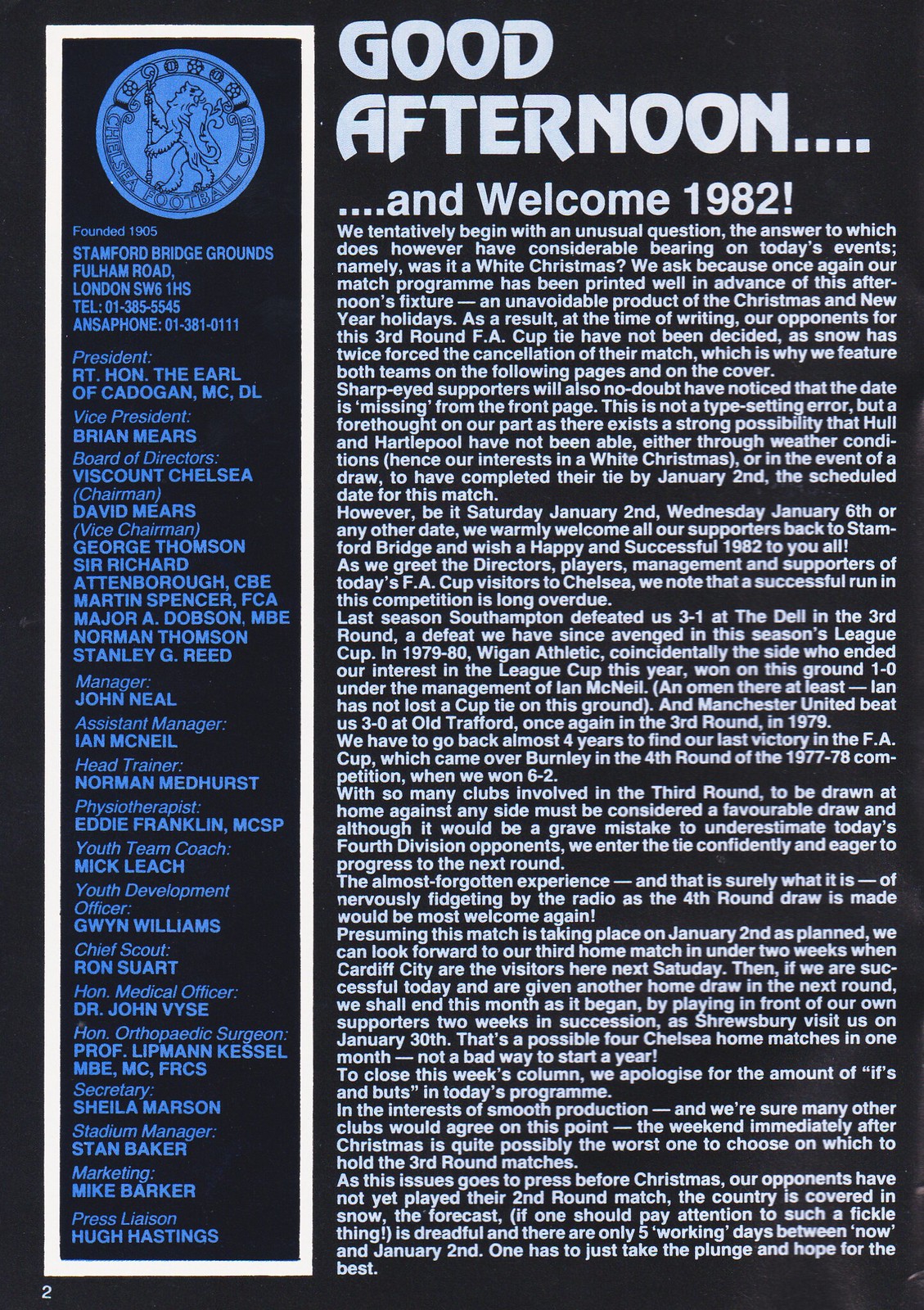The image depicts the second page of a magazine or possibly a web page with a predominantly black background. The layout is divided into two sections. On the left, a thinner column is bordered in white and features a blue circular seal at the top, with a logo depicting a lion holding a bar. Below the seal, text in small print provides details including "Founded 1905" and "Stamford Bridge Grounds, Fulham Road, London," followed by a list of titles and names such as President, Vice President, Board of Directors, Manager, Assistant Manager, and Chief Scout. The main section of the page on the right features a bold white title at the top saying "Good Afternoon.... Welcome to 1982!" Below this greeting, a large body of smaller white text continues, discussing topics related to a sports club, mentioning the FA Cup, matches, and a victory with a score of 6 to 2. The entire page appears to focus on introducing or providing updates from this sports organization, likely set in the context of a historical or commemorative publication.